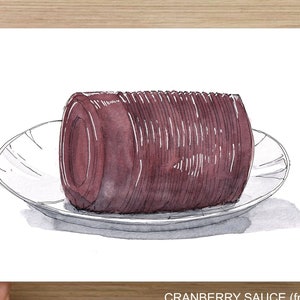A detailed hand-drawn illustration features a gelatin-like, canned cranberry sauce lying on its side atop a bright white, decorative glass plate. The cranberry sauce retains the cylindrical shape and grooved indentations from the can, with a smooth, patchy area at the top and muted red color interspersed with white light reflections. This illustration, rendered on white paper, is framed by light brown wooden panels at both the top and bottom. The square format of the image includes subtle shadowing, and the bottom panel bears the partially cut-off, white-printed text "cranberry sauce," anchoring the whimsical depiction in a cohesive composition.